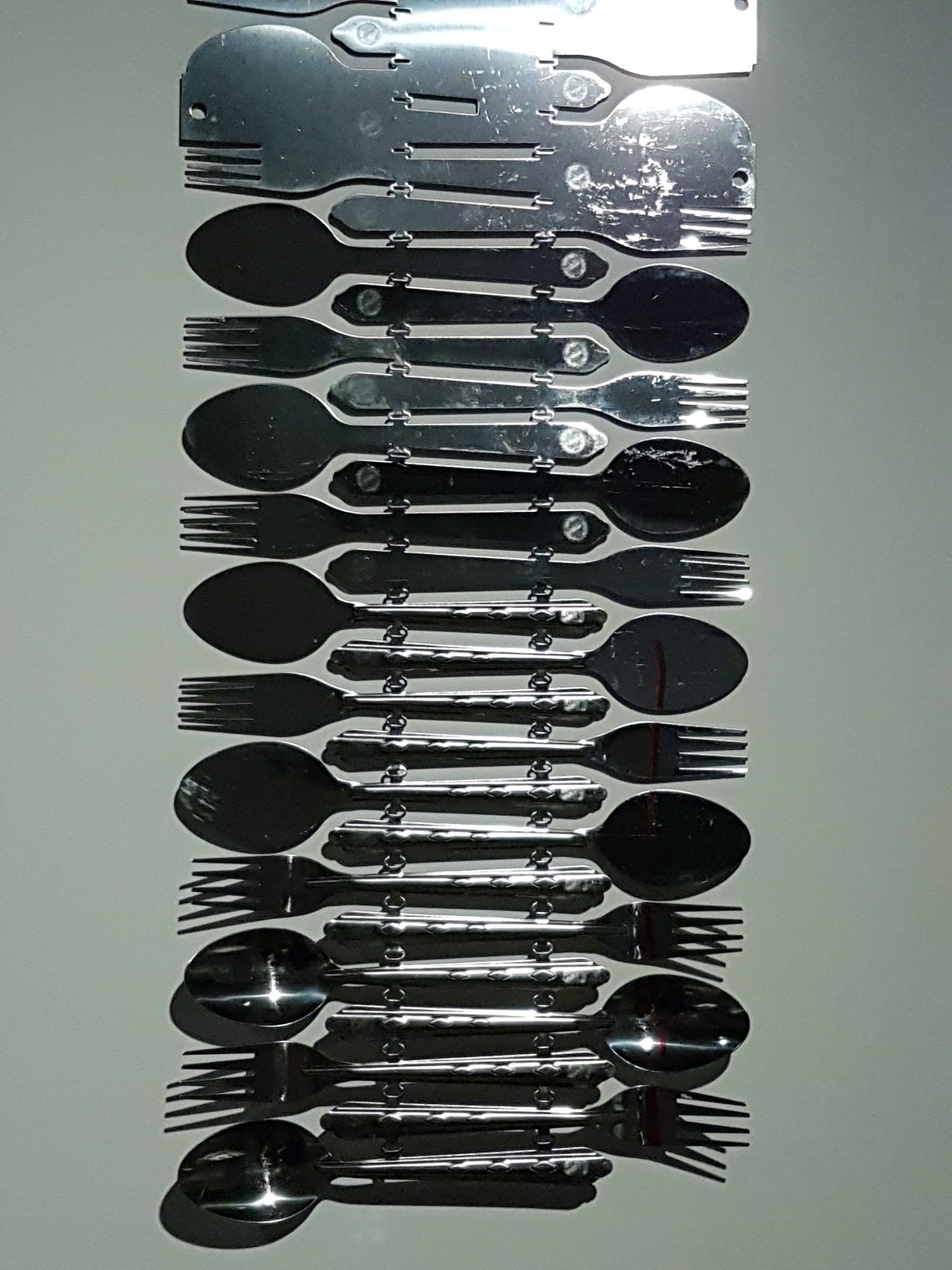This photograph captures a meticulously arranged vertical stack of silverware against a light green background, which gives the illusion of a gray hue. The silver utensils, comprised of spoons and forks, are artfully displayed in an alternating and rhythmic pattern from top to bottom. Each piece faces a different direction: spoons point to the left while forks point to the right. The utensils are consistently aligned with thin handles and four-pronged forks featuring rounded oval-shaped spoon heads. At the very top of the display, the utensils appear to merge together, creating a blended silhouette that adds a unique artistic touch to this structured and visually appealing display piece.